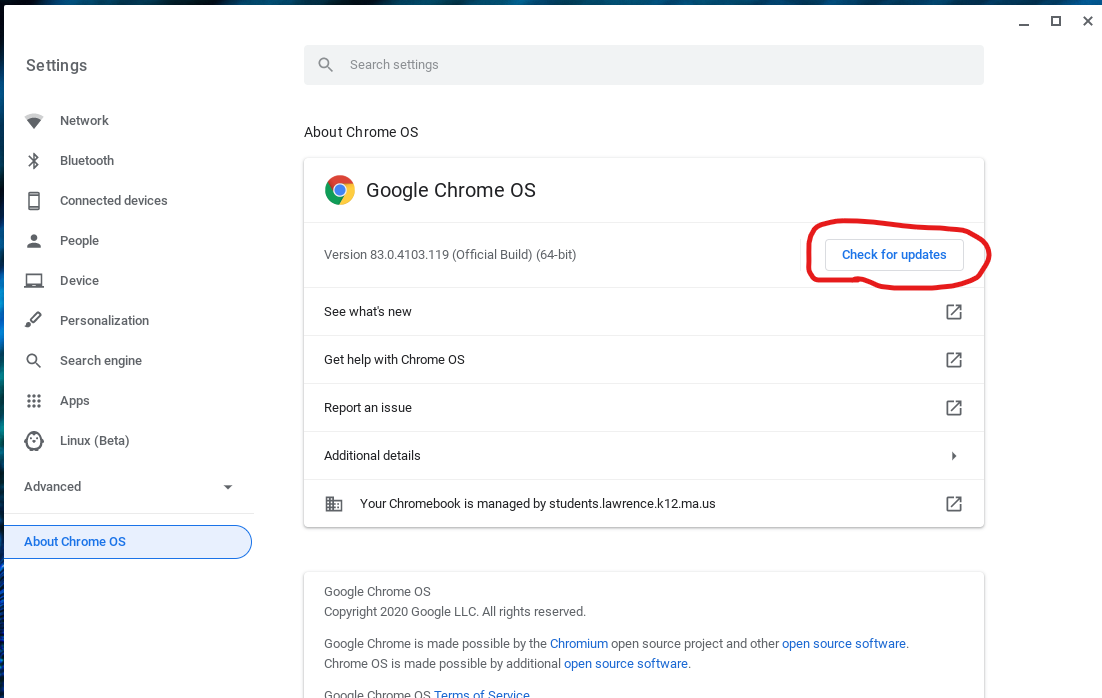The image depicts the settings page of a Google Chromebook, shown in landscape orientation. The interface features a prominent "Search settings" bar at the top.

On the left side, a vertical rectangular section lists various settings categories, including:
- Network
- Bluetooth
- Connected devices
- People
- Device
- Personalization
- Search engine
- Apps
- Linux (Beta)
- Advanced (which is expanded to show additional settings)
- About Chrome OS

In the center of the screen, the "About Chrome OS" section is displayed. At the top, it features the Google Chrome logo alongside the bold text "Google Chrome OS" and the current version number. To the right, a box labeled "Check for updates" is encircled in red, indicating a hand-drawn emphasis, perhaps to guide users on how to update their Chrome OS. 

Below the version number, options include:
- See what's new
- Get help with Chrome OS
- Report an issue
- Additional details

There is a note indicating that the Chromebook is managed by "Students, Lawrence" with a provided school address. Additional legal information is displayed in small text at the bottom.

This detailed visual appears to be an instructional guide on updating the Chrome OS, likely aimed at users of a school-managed Chromebook.